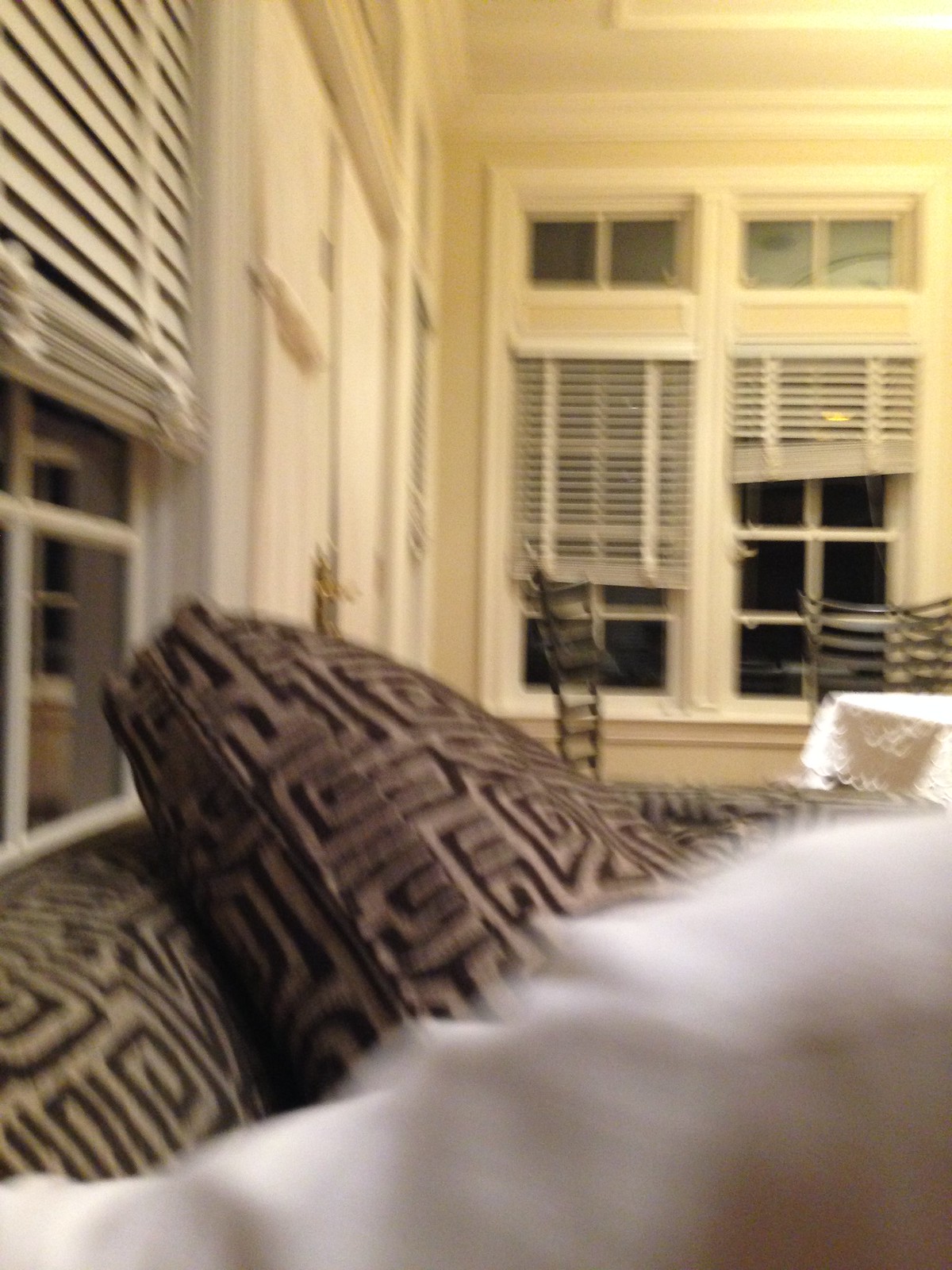In this cozy living room photo, taken from the perspective of someone sitting on the sofa, the foreground features a blurry image of a person's arm adorned in a long-sleeve white shirt. The person is seated on a plush sofa characterized by a dark brown and cream-colored pattern, with one of its cushions flipped up, revealing the zipper on its fabric cover. The sofa is positioned against a window with white frames divided into multiple panes, and the white mini-blinds are partially pulled up, exposing the top pane and a half of the window.

To the right of the scene lies a rectangular table draped in an intricate white lacy tablecloth. It is flanked by two high-back chairs boasting wooden frames and slatted backrests, with one chair pulled up to the table while the other is slightly pulled away. Beyond the table, the room is illuminated by two additional windows, each framed in white and featuring several panes. The mini-blinds on these windows are adjusted differently—one pulled up almost entirely to allow ample light in, while the other is raised just a bit, adding to the room's serene and homely ambiance.